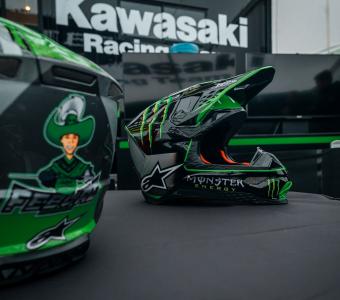The photograph captures two green racing helmets with intricate designs, prominently featuring grey accents and black stars. The leftmost helmet displays an image of a cowboy wearing a cowboy hat, while the rightmost helmet has an open visor, revealing a mostly dark interior with orange lining visible around the edges. The helmets, sponsored by Monster Energy, are strategically placed towards the center of the image on a grey, cushion-like surface. At the top of the image, bold white text reads "Kawasaki Racing," indicating the helmets' association with the brand. In the background, a small patch of grey, overcast sky suggests the photo was taken outside, adding a gloomy ambiance to the scene. The overall color scheme of the image includes shades of green, grey, black, and white, emphasizing its sports racing theme.